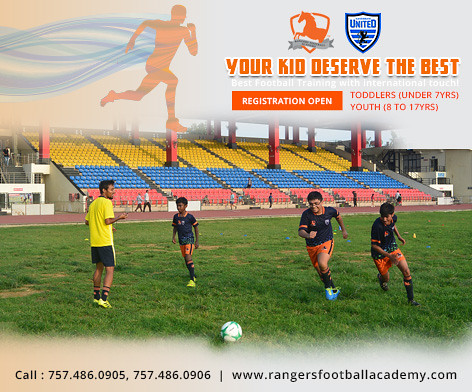This vibrant image captures a dynamic soccer scene showcasing a group of children playing soccer on a lush green field inside a stadium. The kids, dressed in dark blue jerseys with orange accents and black t-shirts with orange shorts, are energetically chasing after a soccer ball. To their left, a coach in a yellow and black outfit observes the action. The stadium seats in the background are striped in pink, blue, and yellow but remain empty, indicating a practice session.

Prominent text overlays the top right corner of the image. In bold, orange, all-capital letters, it reads: "YOUR KIDS DESERVE THE BEST." Directly beneath, white text declares: "Best football training with international touch." A dark orange rectangle below this text announces: "REGISTRATION OPEN," and specifies, "Toddlers under 7 years and Youth, 8 to 17 years." At the bottom of the image, contact information is provided with two phone numbers: "757-486-0905, 757-486-0906," and a website: "www.rangersfootballacademy.com." Additionally, the top left corner features a stylized graphic of a person running with motion trails. This cohesive advertisement promotes exceptional football training opportunities for children, emphasizing accessibility and quality.